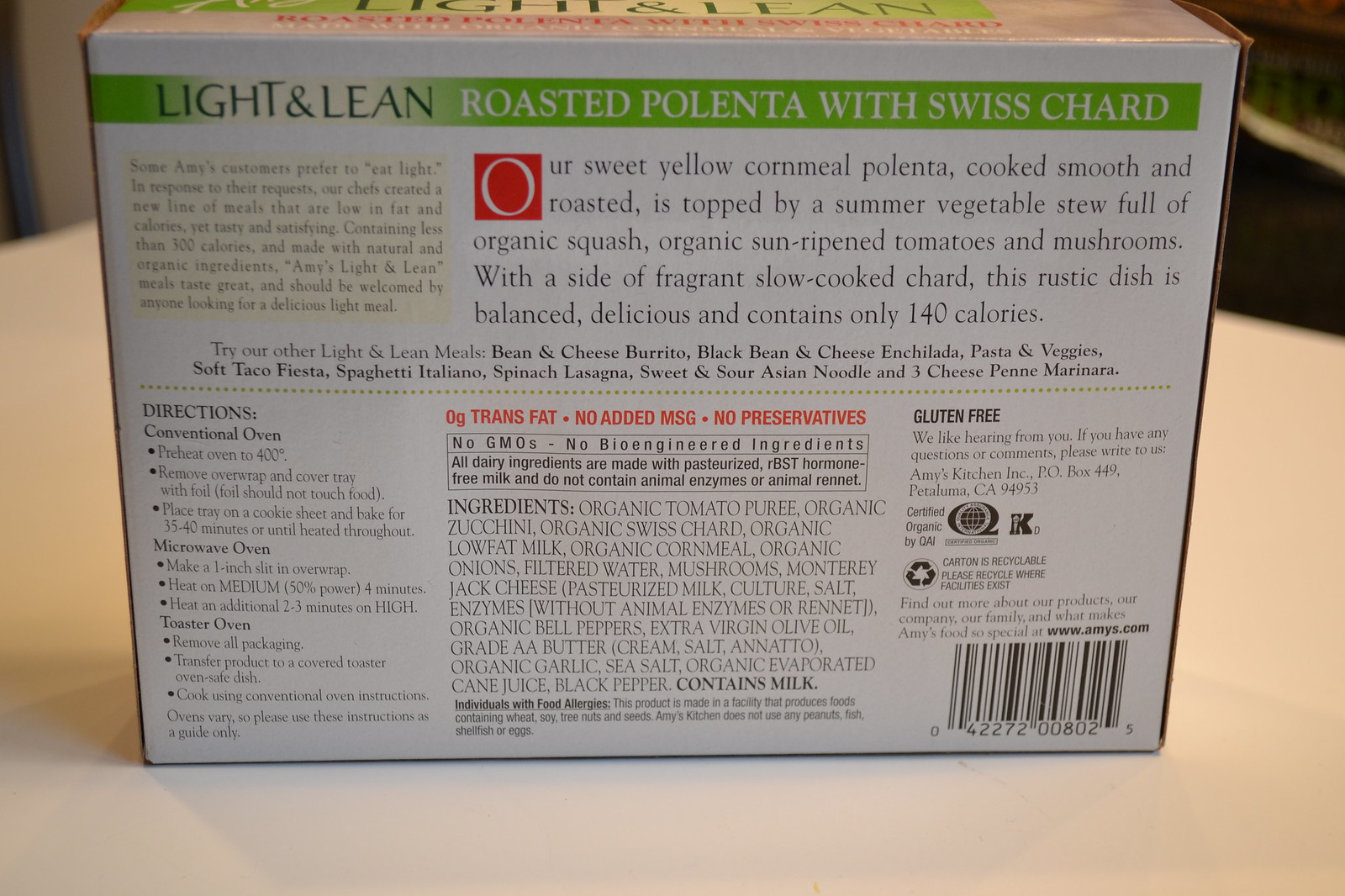This landscape-oriented color photograph captures the back of a rectangular cardboard food box, presumably taken in a kitchen with central lighting. The box, standing on its longest side, is positioned on a white, round table or counter. The packaging prominently features a green strip across the top that reads "Light and Lean" in black letters and "Roasted Polenta with Swiss Chard" in white letters. Below this, detailed product information is displayed, describing the dish as sweet yellow cornmeal polenta, cooked smooth and roasted, and topped with a summer vegetable stew containing organic squash, organic sun-ripened tomatoes, and mushrooms, served alongside fragrant, slow-cooked chard. Additional information includes directions for preparing the dish in a conventional oven, microwave, or toaster oven, nutritional content, ingredients, and a barcode in the bottom right corner. The packaging also highlights key features in small red font, noting it contains zero trans fat, no added MSG, and no preservatives. The product is characterized as balanced, delicious, and containing only 140 calories, and is identified as gluten-free.